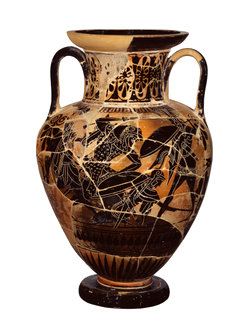The image is a color photograph in portrait orientation, showcasing an ancient urn or vase set against a pristine white background, appearing to float in space. The vase has a classical tapered design with a wider body at the shoulders, a narrow neck flaring out at the top, and a circular foot at the bottom. It features two handles—one on each side near the top—connecting to the widest part of the vase.

The vase predominantly exhibits dark bronze and brown tones. Its surface is adorned with intricate imagery, primarily in black, accented with white lines, set against an orange-brown background. These illustrations depict figures reminiscent of ancient Greek mythology, including soldiers with large shields and mythological creatures, some bearing animal-like heads. The figures are highly detailed, suggesting a Dionysian theme common in Greek art, despite the paint showing signs of age with cracks and chips, hinting at its archaeological restoration. The overall photographic style is one of representational realism, capturing the fine details and textures of the ancient vase.